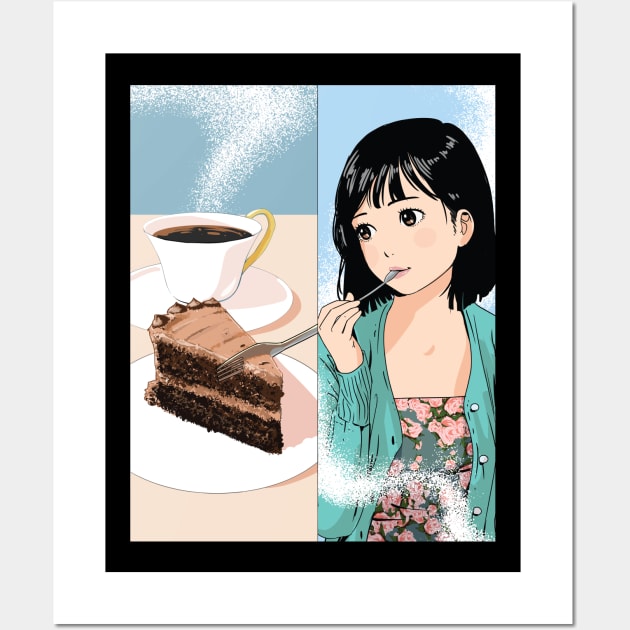The image features a detailed digital artwork styled like a comic book or manga, with a light and airy watercolor feel. The piece is presented within a picture frame that has a white outer border and a black inner border, hung against a light gray wall. The composition is divided into two panels by a thin black line.

On the left panel, there is a depiction of a double layer chocolate cake on a white platter, with a fork poised to take the first bite. Behind the cake, a steaming cup of coffee sits on another white plate, both set against a blue-toned background.

The right panel showcases a young woman of Japanese descent with shoulder-length dark hair and bangs, who is wearing a green button-up long-sleeve shirt over a teal blue flower-patterned crop top. She has fair skin and large brown eyes. The woman, with a joyful expression, has a fork in her mouth and seems to be gazing thoughtfully towards the cake, embodying a moment of daydreaming or deep contemplation. This cohesive and vibrant scene captures the essence of indulgence and introspection.